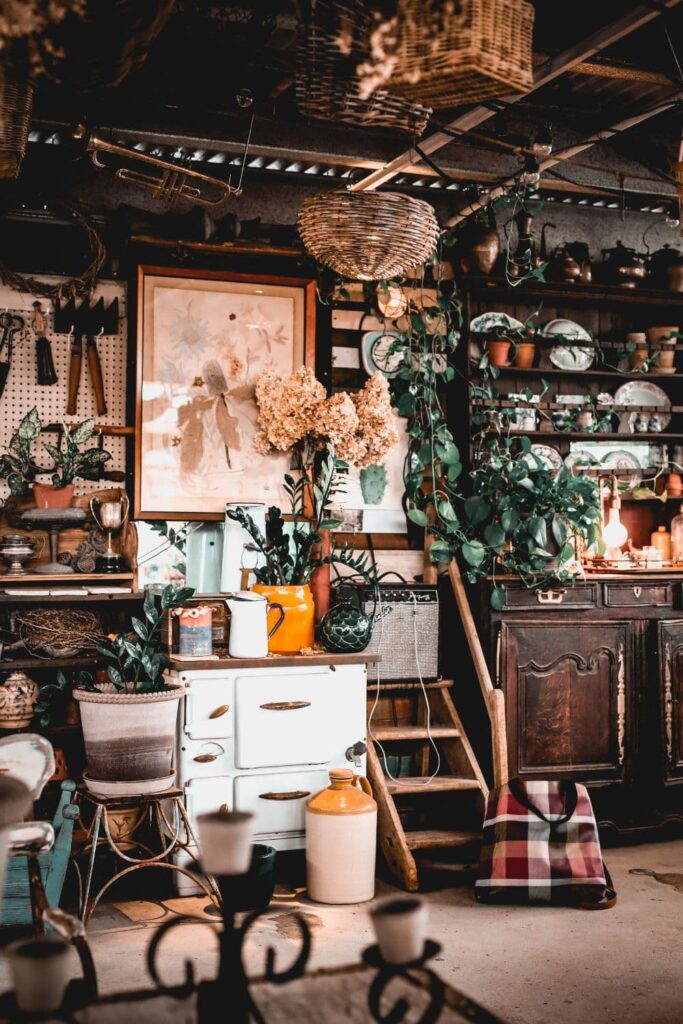The image depicts the interior of a charming antique store, exuding a warm and nostalgic wooden ambiance. Diverse items crowd the space, with numerous vintage wooden desks and armoires adding to the timeless allure. Dominating the scene is a central desk, primarily white, which immediately draws the viewer's attention. Atop the white desk sits an elegant white kettle, a distinctive brownish-red and blue can, and a classic Fender guitar amplifier. The amalgamation of these carefully curated antiques and musical equipment creates an eclectic yet harmonious setting, captivating anyone who steps into this treasure trove of bygone eras.